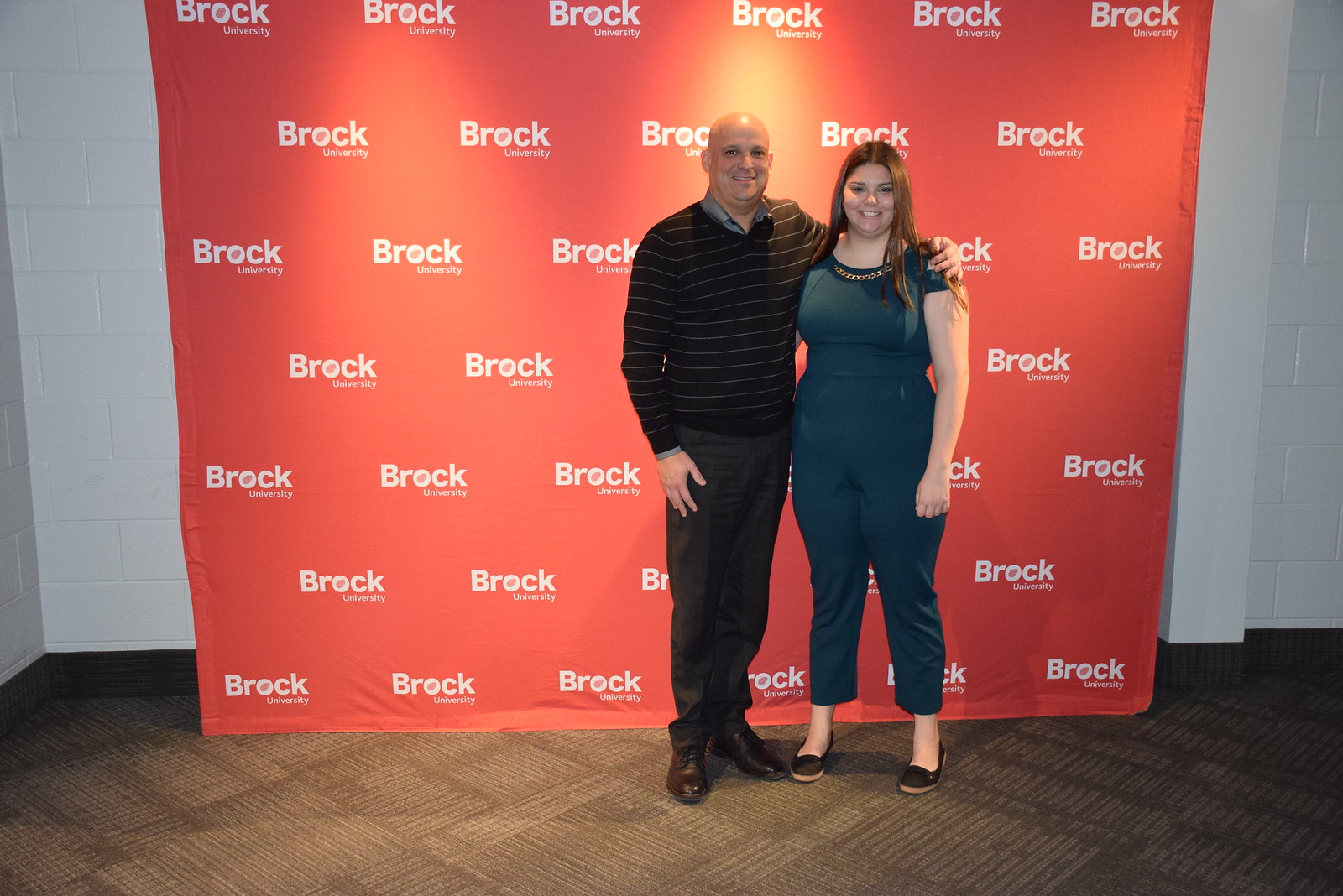This is a detailed photograph of a man and a woman standing slightly to the right of center, in front of an orange backdrop repeatedly emblazoned with "Brock University." The setting has a tan carpeted floor. The bald man, on the left, is dressed in a black and white striped sweater with a gray collared shirt underneath. He pairs this with black dress pants and black shoes. His right arm lovingly drapes over the woman's shoulder, while his left hand rests at his waist. The woman, standing to his right, has long dark hair that falls just past her shoulders. She is adorned in a steel blue outfit consisting of a short-sleeved top with a gold chain necklace and matching blue capris that end a few inches above her black shoes. Both individuals are smiling warmly at the camera, exuding happiness and contentment.